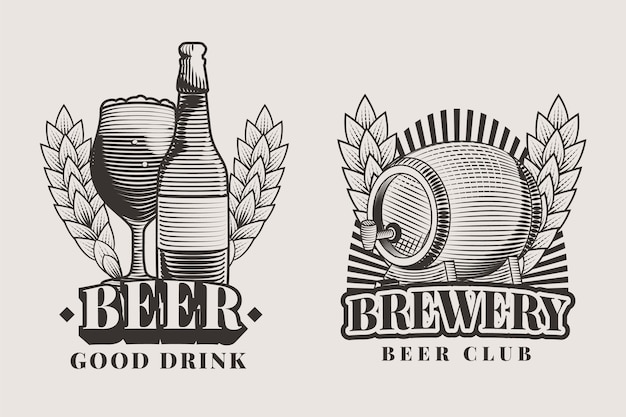The placard, predominantly in black and an off-white color scheme, serves as an advertisement for a beer club. The background is a light grey that complements the detailed black and greys of the artwork. On the left, the text "Beer, Good Drink" is displayed alongside an image of a beer bottle with horizontal stripes and a glass brimming with foam, indicative of the beer's head. Surrounding the bottle and glass are decorative elements resembling hops or grains, adding a natural flair. On the right side of the placard, a cask with a tap sits on a stand, adorned similarly with hops or grain decorations. Below the cask, the words "Brewery Beer Club" are inscribed, anchoring the advertisement's purpose. The overall design is accentuated with black lines and stylized grain motifs, creating a cohesive and inviting visual appeal.